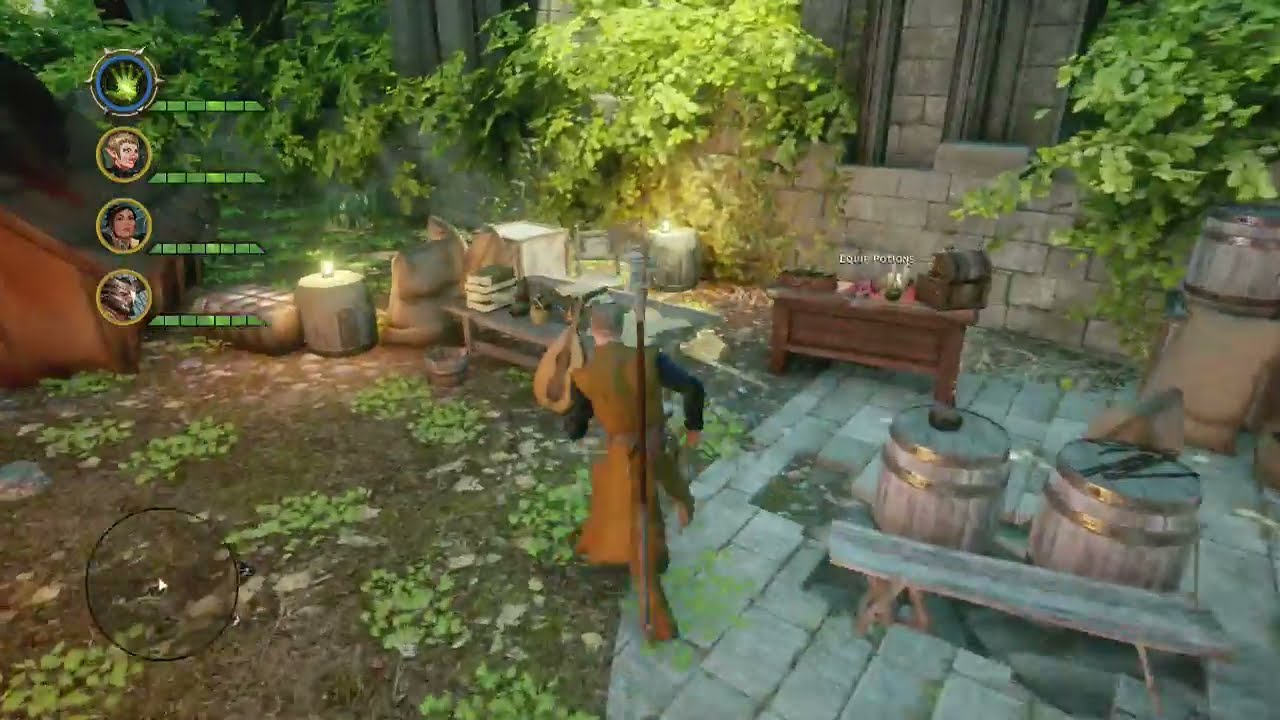This is a detailed screenshot from a 3D video game, showcasing a richly decorated room with a mix of classical and fantastical elements. In the upper left corner, there are three character icons with corresponding health bars. One icon features a green hand, while the others depict characters including one with light skin and yellow hair, another with white skin and dark hair, and a third resembling a werewolf. These health bars display various levels of green and red, indicating remaining health.

The ornate room itself features a mix of marble and tiled flooring, with a multicolored rug in the center. The walls are a shade of gray and adorned with paintings in golden frames, one showing a brown walkway and another with a white sculpture. Marble statues, golden figurines, small treasure chests, and an ornate cup add to the room's lavish decor. In the far right corner stands a knight holding a shield, while yellow columns support the ceiling. Beige curtains with red designs hang from the walls, and a radar map in the bottom left corner guides the player. The scene is incredibly detailed, almost photorealistic, capturing an old-century ambiance fused with fantasy elements.